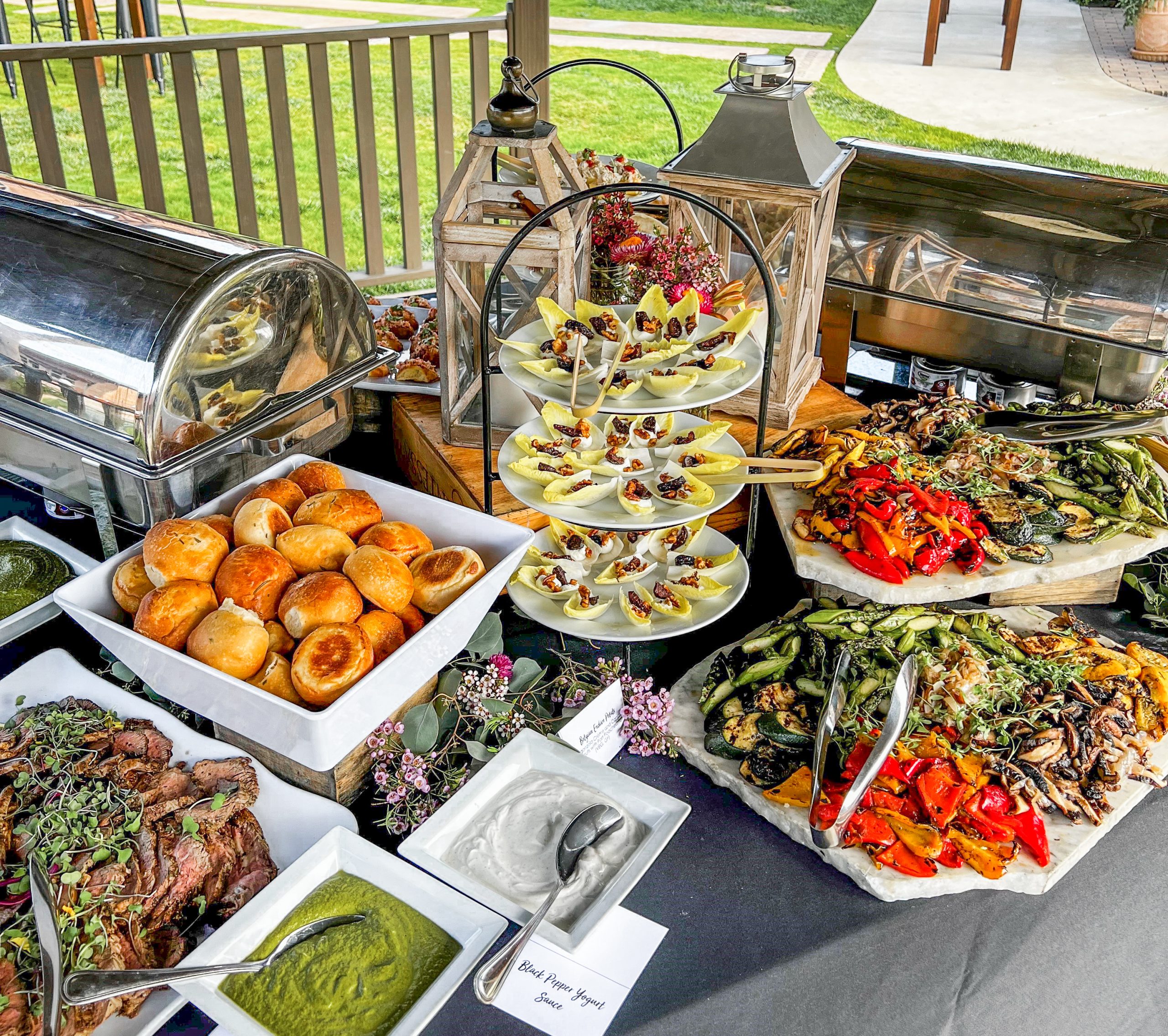This detailed photo captures an elaborate outdoor food spread, seemingly set up either in a backyard, park, or deck area, where the background features wooden fencing, concrete walkways, and grassy patches. The focal point is a large table draped in a gray tablecloth, adorned with an impressive array of dishes and culinary delights. The spread includes various types of meats, bread rolls, and grilled vegetables. White serving dishes overflow with colorful offerings, accented by utensils such as tongs, spoons, and forks for easy serving.

Notably, there are two buffet-line containers with stainless steel, domed lids designed to keep the food warm. Accompanying the main dishes are green and white sauces likely to be guacamole and sour cream, respectively. The table also displays several stacked platters featuring what appear to be artichoke leaves or lettuce wraps filled with hors d'oeuvres, perhaps oysters or nuts in sauce.

Adding to the aesthetic, unlit wooden and metal lanterns are placed along the table, enhancing the welcoming atmosphere. Overall, the scene is beautifully set, suggesting an inviting and sumptuous outdoor dining experience.